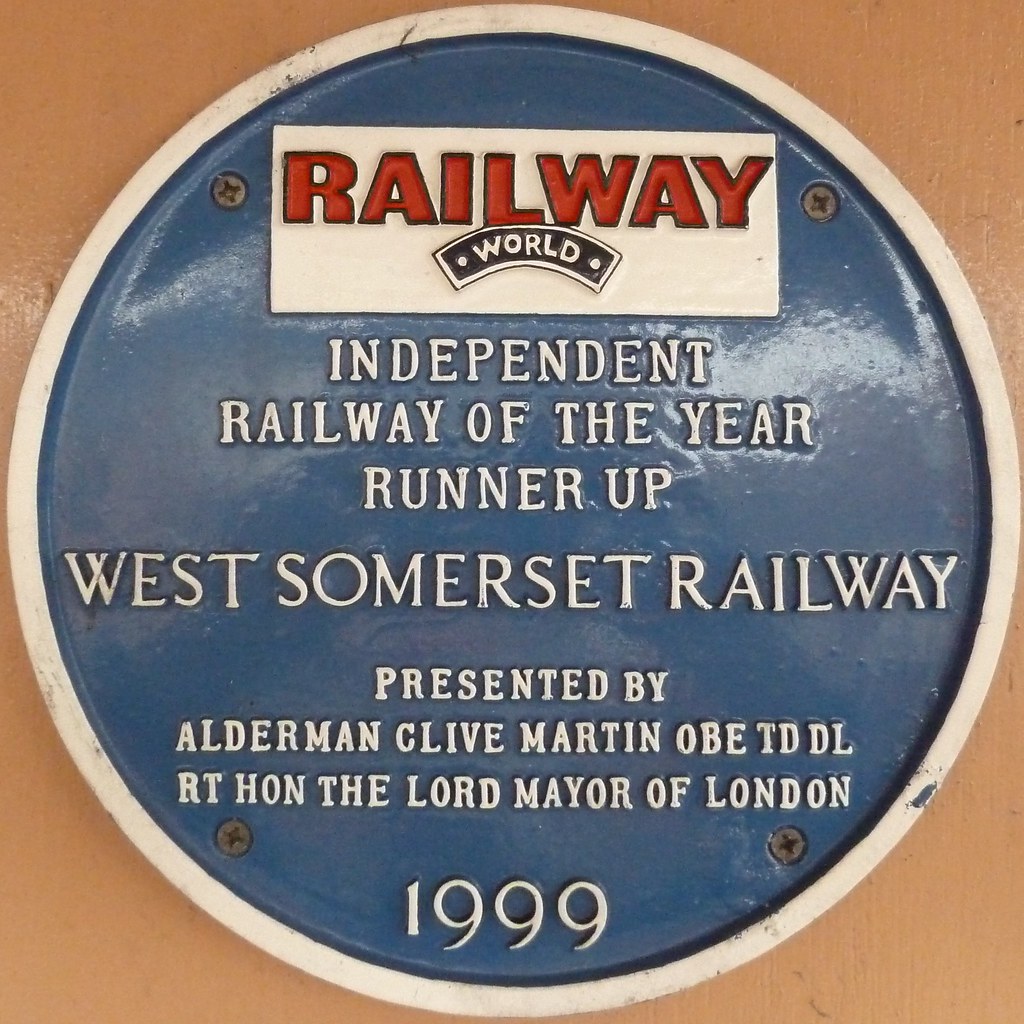The image depicts a glossy, circular metal sign firmly screwed into a wall of a light brown, dark peach, or tan color. The sign, which appears to have a ceramic coating, features a prominent blue center encircled by a white border. At the top of the blue circle, a white text box with red lettering reads "Railway World." Below this, in white letters on the blue background, the text states, "Independent Railway of the Year Runner-Up, West Somerset Railway." The sign also notes that it was presented by Alderman Clive Martin, OBE, TD, DL, RT Hon, the Lord Mayor of London in 1999.